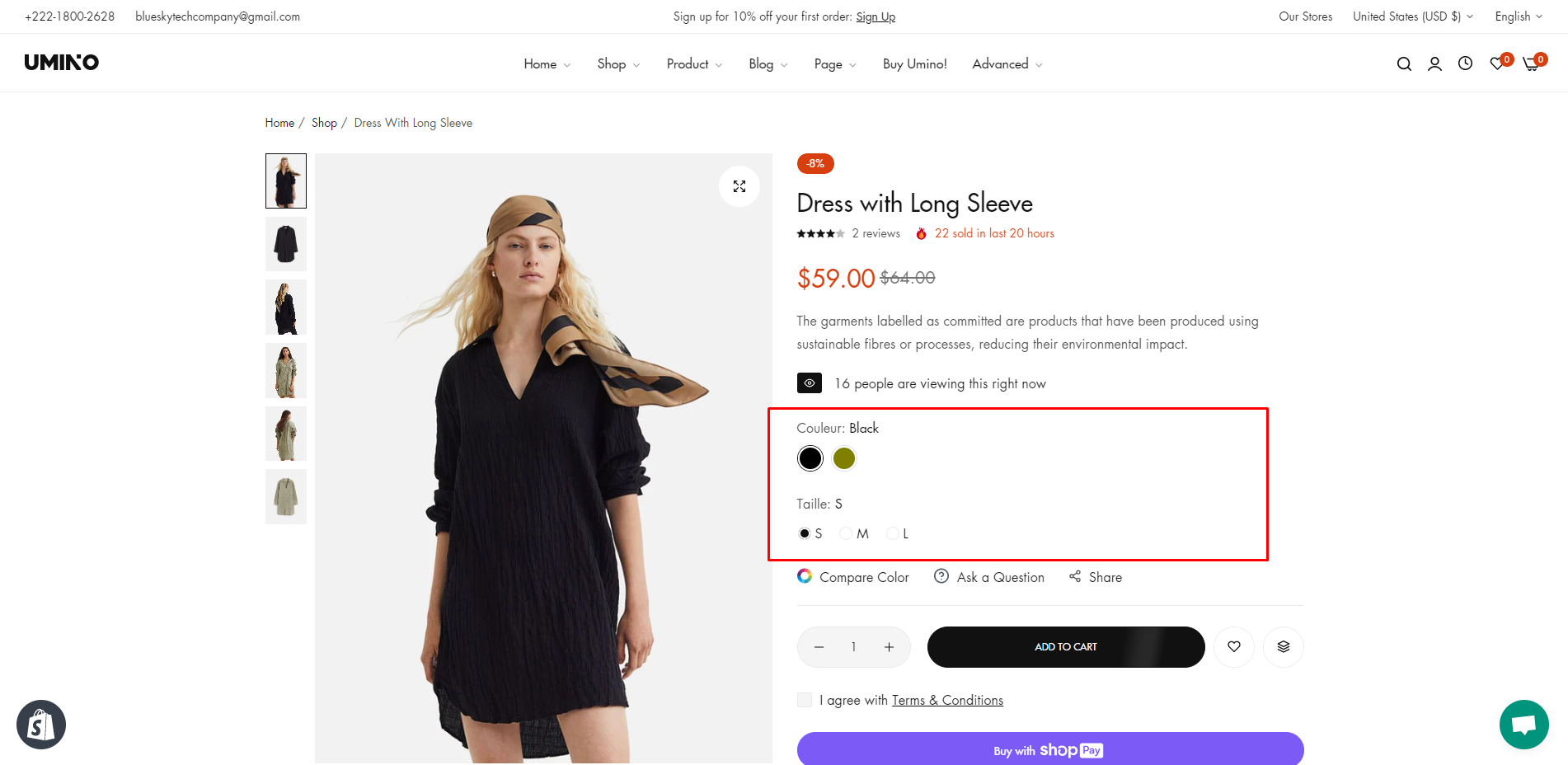On a predominantly white background, this image features black text positioned in the upper left corner. The text includes a generic phone number, "+222-1800-2628," and an email address. Centered on the image in bold black text, it proclaims, "Sign up for 10% off your first order," with the word "Sign up" underlined.

In the upper right corner, the text reads: "Our Store," "United States," represented by a U.S. flag icon, "U.S. Dollar" indicated by a dollar sign symbol, and "English." Below this section is the company's dark black logo with the text "U.M.I.N.O."

Spanning the center area of the image is the website's main navigation bar, listing options such as "Home," "Shop," "Products," "Blog," "Page," "myUMO," "Advantage!" Additionally, on the right side of the navigation bar, there are icons for a magnifying glass (search), a person (account), a clock (possibly for quick access or history), a heart (favorites or wishlist), and a shopping cart.

Below the navigation bar, a striking image of a woman wearing a hippie-style tan headscarf with black patterns and a stylish black dress is centered. She has white-blonde hair and is looking directly at the camera. On the left side of the dress, various styles of this outfit are displayed.

To the right of the woman's image, there is a description of the dress, titled "Dress with Long Sleeve," accompanied by two reviews with a four-star rating. The dress is priced at $59, highlighted in red text. Below the price, there is a red selection box for color options, offering choices between black and a greenish-tan color.

At the bottom of the image, there is a blue-outlined box with white text that reads, "Buy with Shop Pay."